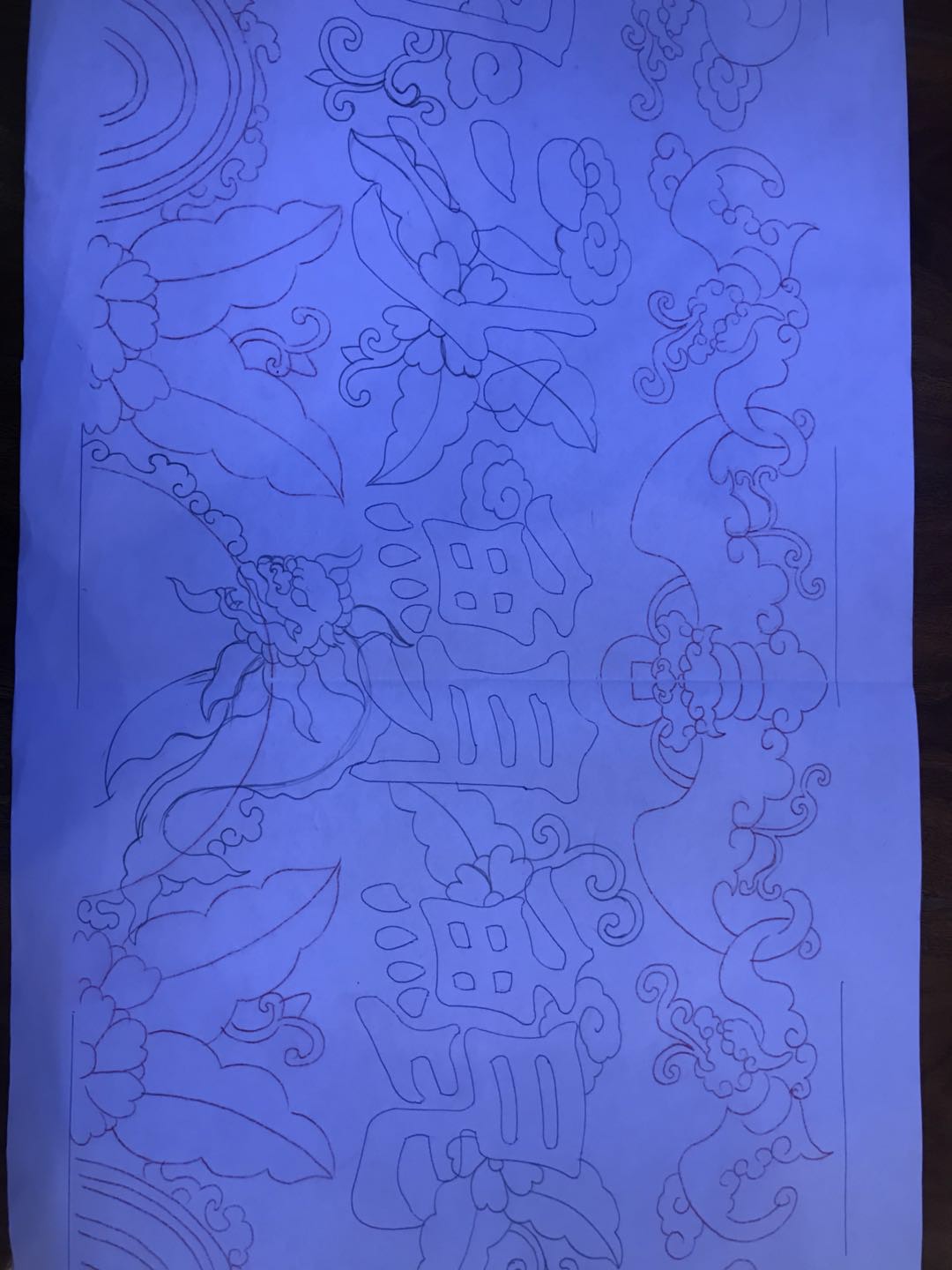This is a detailed, black and white pencil drawing on a piece of paper that appears purple and has a slight crease in the middle. The drawing is oriented vertically but is meant to be viewed horizontally. The composition is intricate and filled with numerous curving lines and overlapping elements. 

In the upper left-hand corner, a series of double-lined half circles create a rainbow-like pattern. Below this, on the left side, are two prominent leaves, followed by another half-circle below them. This half-circle forms the head of a dragon, featuring an open mouth with visible teeth and a mane-like structure around its head. Surrounding the dragon are various leaves and flower petals. Above the dragon's head, delicate and flowing designs of curves and curls stretch across the top of the image, adding to the complexity.

In the center of the drawing, several squares and rectangles are arranged, some containing smaller squares or rectangular shapes within them, though their meaning remains ambiguous. Interspersed throughout the image are additional leaves and floral elements, blending into the abstract design seamlessly. Above these geometric shapes, what appear to be outlines of Asian characters can be seen, layered with more leaves and flowers behind them. The overall effect is a rich tapestry of shapes and forms that come together in a detailed and captivating scene.